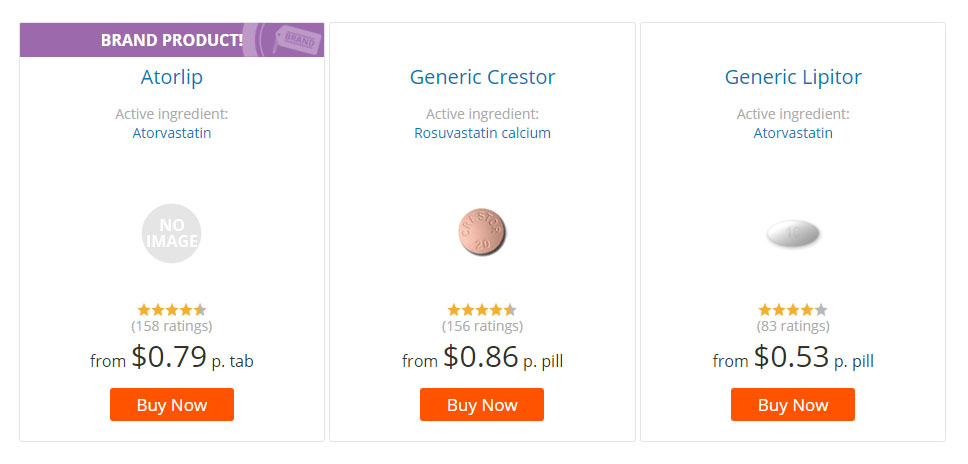Detailed Caption:

This is a screenshot of a pill identifier or drug information website. The page prominently displays three distinct pill panels in a simple layout, without any headers or footers. Each panel provides detailed information about a different medication.

1. **Ator Lip**:
   - **Active Ingredient**: Atorvastatin
   - **Pill Appearance**: Gray, round, no specific pill image available.
   - **Price**: Starts at 79 cents per tab.
   - **Action Button**: Orange "Buy Now" button is present for purchasing.

2. **Generic Crestor**:
   - **Active Ingredient**: Not mentioned specifically, but implied to be similar to Crestor.
   - **Pill Appearance**: Small, round, reddish pill.
   - **Price**: 86 cents per pill.
   - **Action Button**: Similar orange "Buy Now" button as in the first panel.

3. **Generic Lipitor**:
   - **Active Ingredient**: Atorvastatin
   - **Pill Appearance**: White, lozenge-shaped pill.
   - **Price**: 53 cents per pill.
   - **Action Button**: Orange "Buy Now" button identical to the other two panels.

Each panel consistently uses a similar layout and design, offering users a clear and concise comparison of the featured medications.